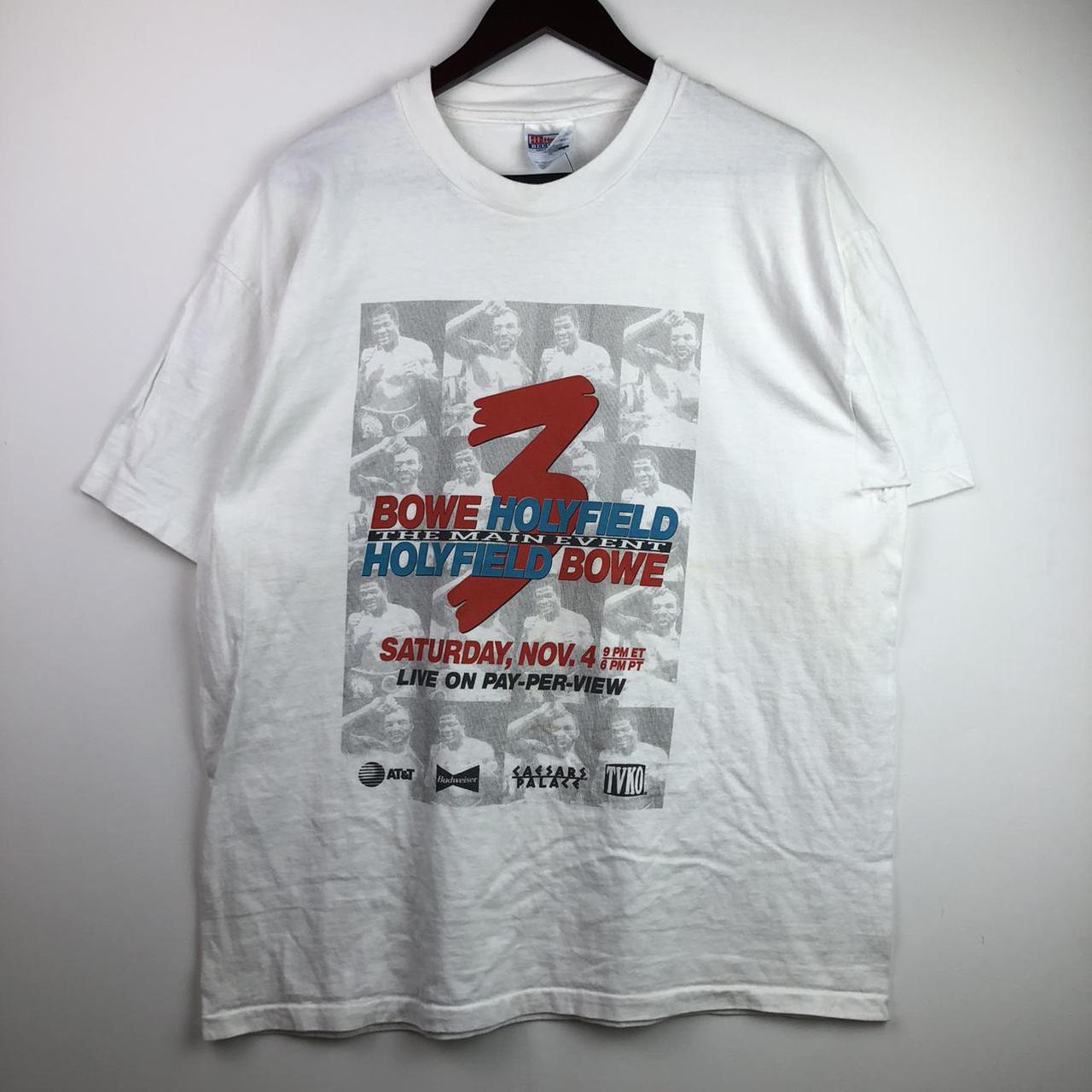This photograph features a slightly wrinkled, vintage white t-shirt hanging on a black hanger against a white-gray wall. The shirt showcases a graphic promoting a boxing event, predominantly illustrated with black and white images of boxers as its backdrop. Prominent in red text is the number "3," along with the names "Bowe" and "Holyfield." Additionally, it reads "The Main Event" between the names. Details include "Saturday, November 4th" and the time "9pm ET, 6pm PT" also specified. It mentions "Live on Pay-Per-View" in blue text. At the bottom of the shirt, there are various corporate logos including AT&T, Weiser, Caesars Palace, and TV KO. Overall, the lighting in the image is dim, emphasizing the thrifted or second-hand nature of the garment.